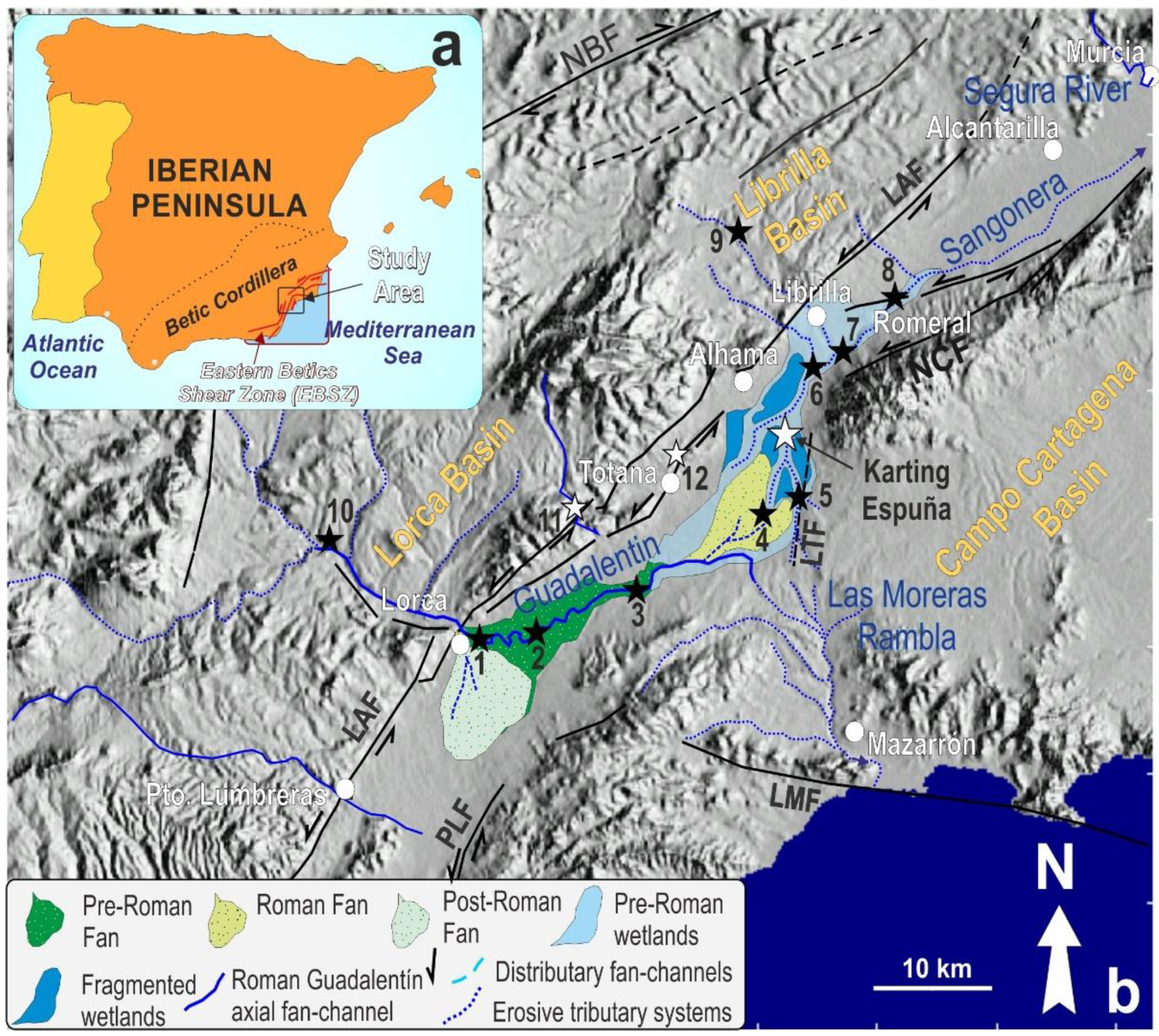This detailed photograph presents a meticulously rendered map of the Iberian Peninsula, prominently displaying Portugal and Spain. The top-left corner features an inset map, helping viewers locate the Iberian Peninsula within a broader geographical context. The main section offers a close-up view of this region, with the land depicted in grey tones and textured regions marking mountainous or elevated areas. In the bottom right corner, the deep navy blue color represents the surrounding sea. 

A comprehensive legend occupies approximately three-quarters of the bottom left region, detailing various features such as different types of wetlands. The map is richly annotated with text in multiple colors—yellow, blue, white—as well as black and white stars and black numerical markers, providing a wealth of information about the geography and topography of the Iberian Peninsula.